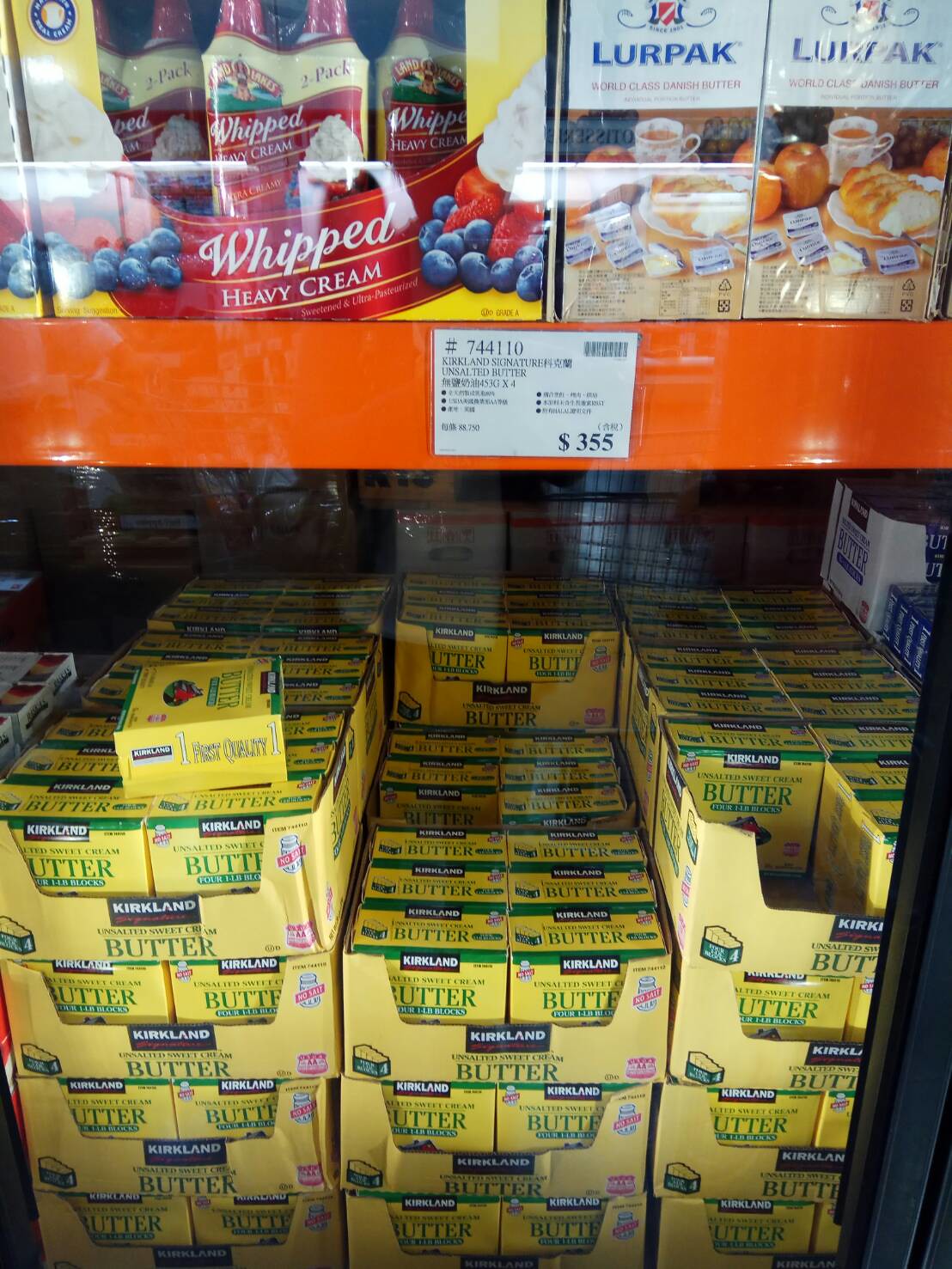This image depicts the freezer section of a Costco store. Dominating the bottom shelf are large stacks of Kirkland Signature unsalted butter, which comes in yellow boxes adorned with prominent green lettering that reads "butter." Each box also features the Kirkland Signature logo, which is black with white and red text. Above this section, there is an orange-colored shelf bearing a white label. This label displays the number 744110, a barcode, and a price of $3.55 beside the product name "Kirkland Signature unsalted butter," though the remainder of the text is not legible. The shelf appears to be in a glass-covered freezer. Above this butter display, on the upper shelf, there are boxes containing cans of whipped cream, which are colored in yellow and red. Adjacent to these, on the left, are boxes of Lurpak Danish butter, recognizable by their white and blue design with images of bread and butter at the bottom.